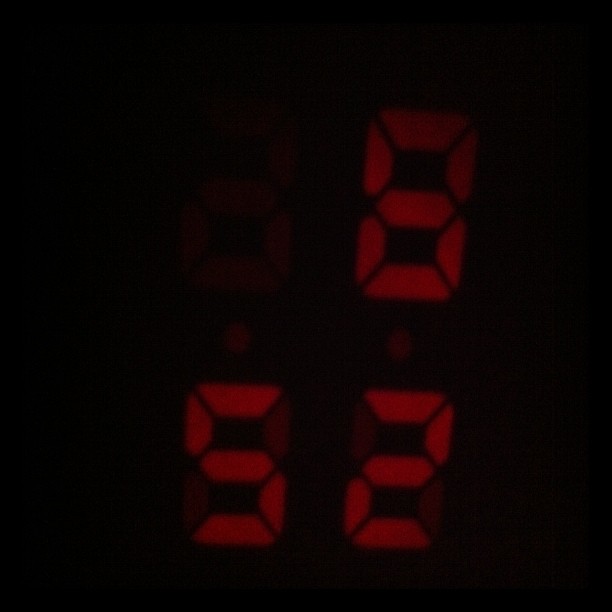A digital clock displays the current time as 8:52, with the hour positioned above the minutes. The clock is square-shaped, and although you can faintly see the image of the preceding hour digit, the display prominently shows the current time. The numbers, rendered in a boxy, segmented style with visible lines at each joint where the segments begin and end, are red and somewhat faded, making them difficult to read clearly. The red digits contrast against a black background, which blends seamlessly into the surrounding black, obscuring the edges of the clock. Additionally, faint dots are present between the hours and minutes, adding to the overall confusing appearance of the display.